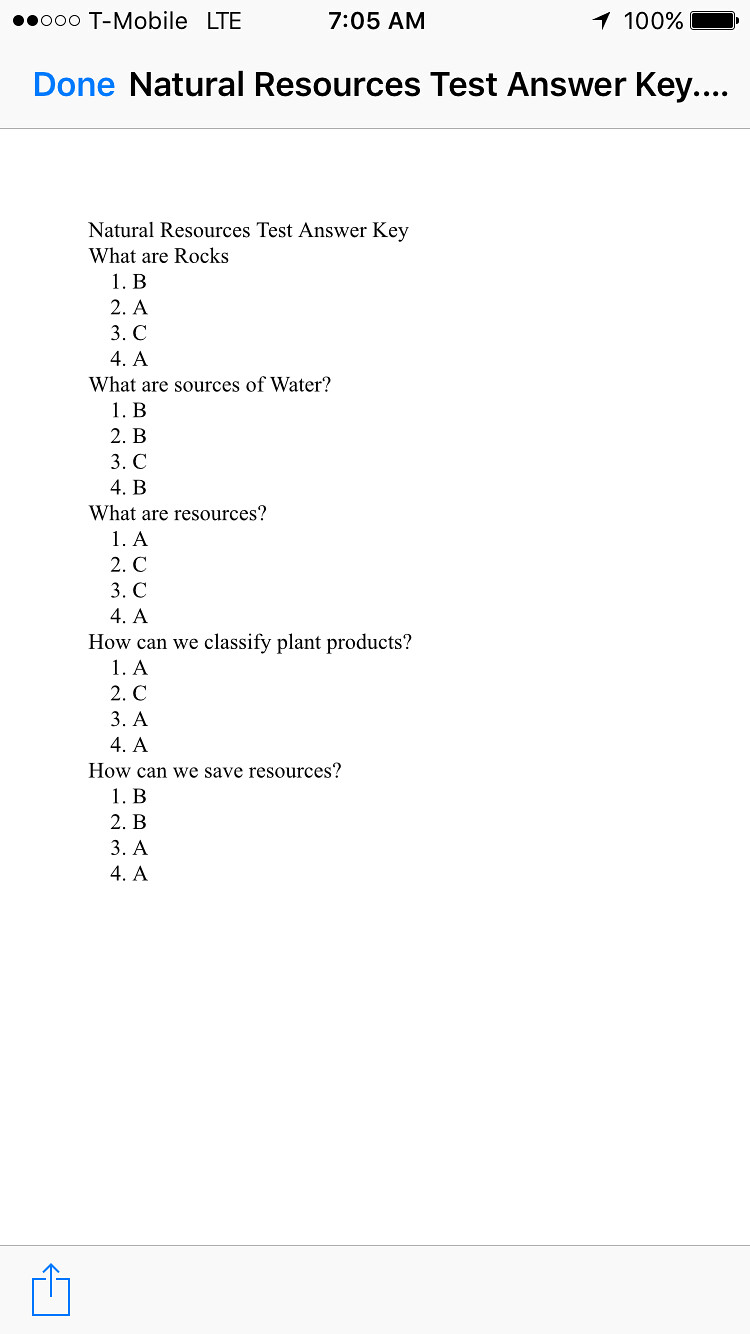The image is a screenshot taken from a smartphone, likely an iPhone, as indicated by the user interface at the top. At the very top, five signal bars are displayed, with only two of them illuminated, suggesting moderate signal strength. The service provider is T-Mobile, the network is LTE, and the time shown is 7:05 AM. On the right side, a triangular icon, tilted approximately 60 degrees, accompanies a fully charged battery icon displaying 100%.

Below this top bar, the screen shows a blue text, "Done," and beneath it, in black text, the header reads, "Natural Resources Test Answer Key…” followed by an ellipsis. The answer key lists five questions related to natural resources, each followed by multiple-choice answers labeled A, B, or C.

The questions and their corresponding answers are:

1. What are rocks?
   - 1. B
   - 2. A
   - 3. C
   - 4. A

2. What are sources of water?
   - 1. B
   - 2. B
   - 3. C
   - 4. B

3. What are resources?
   - 1. A
   - 2. C
   - 3. C
   - 4. A

4. How can we classify plant products?
   - 1. A
   - 2. C
   - 3. A
   - 4. A

5. How can we save resources?
   - 1. B
   - 2. B
   - 3. A
   - 4. A

Each set of answers contains four numerical options, broadly spread across different choices. The screenshot's meticulous details and structure confirm that it is meant for educational purposes, specifically serving as an answer key for a test on natural resources.